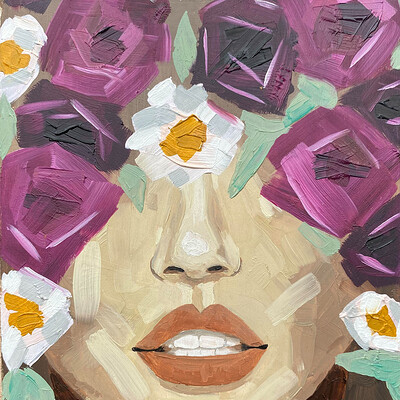In the image, a square-shaped painting, likely created using oil or fabric techniques, showcases a woman's face prominently positioned in the lower center. The visible parts of her face include a slightly open mouth with revealed white teeth and red lipstick, while her eyes are obscured by an array of flowers. The background features textured paint designed to mimic floral patterns. The flowers include light and dark purple roses placed on both sides, along with scattered white flowers with yellow centers. Additionally, green spots suggest leaves amidst the flowers. The composition includes notable flower placements—one in the middle, another in the top left corner, and others in the bottom left and right corners. The painting employs a limited but elegant color palette, adding to its artistic appeal.